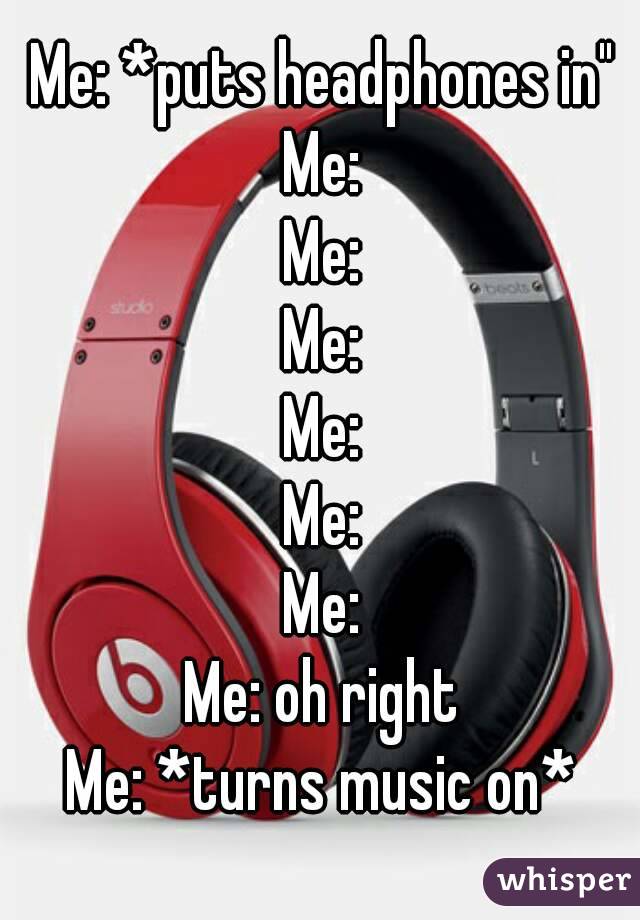This is a detailed image of a pair of over-the-ear Beats headphones, predominantly red on the outside with black padding on the inside for comfortable listening. The headphones are set against a white background, and the red earcups prominently feature a glossy symbol that resembles either a stylized "b" or the number "6," likely part of the Beats branding.

Overlaying the image, there is text formatted in a series of humorous, meme-like statements. At the top, in white font with a black outline, it says, "Me: *puts headphones in*". Below this, running down the center of the image in several rows, there is a repeated "Me:" with no additional text, humorously suggesting a moment of inertia or inactivity. Finally, at the bottom of the image, it concludes with, "Me: *turns music on*," indicating the realization that the user forgot to play the music after putting the headphones on. In the bottom right corner, written in white font within a pill-shaped purple box, is the word "Whisper," possibly indicating a brand or a subtle watermark.